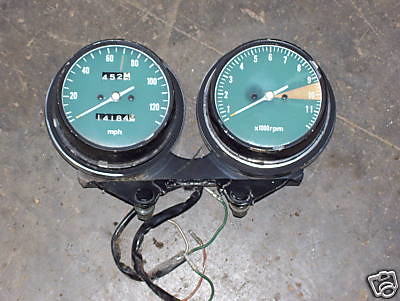This photograph showcases a dual gauge set that appears to be removed from a motorcycle. On the left side, the speedometer displays miles per hour with a striking blue face and crisp white lettering. The analog odometer reads 14,184 miles, with the trip meter showing 452 miles. The right side features a tachometer measuring engine revolutions per minute (RPM), indicating a high-performance engine with a range reaching from 1,000 up to 11,000 RPM. The redline starts at 10,000 RPM, emphasizing the engine’s high capabilities. The gauge assembly has been detached, leaving the wiring harness visible. The background consists of a slightly scarred concrete surface, adding texture to the scene. Additionally, there’s a faint watermark of a camera icon positioned at the bottom right corner of the image.